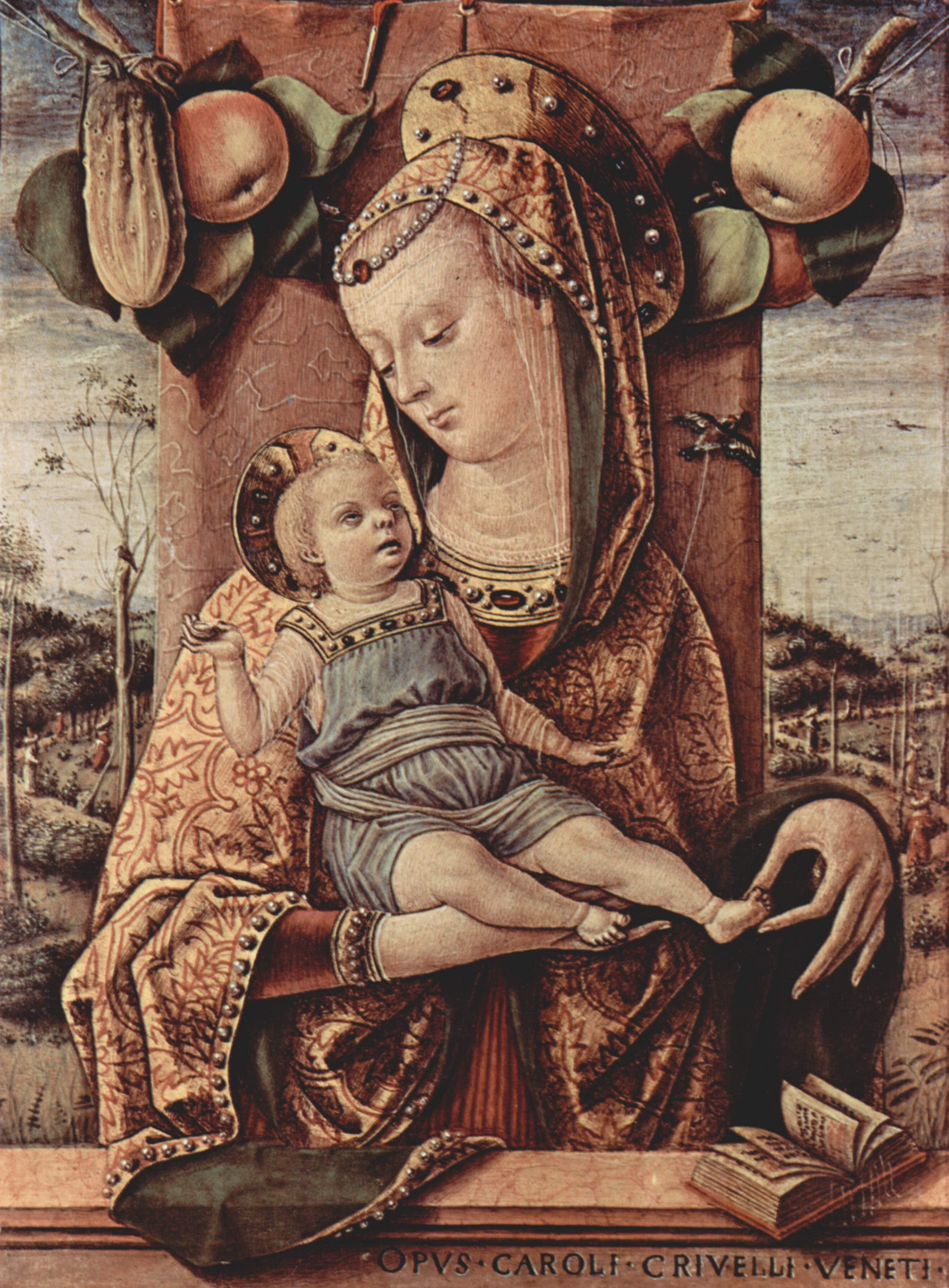In this intricate painting, an elegantly dressed woman, possibly of noble or royal status, is depicted holding a young child. The woman's attire features a golden peach-colored, richly adorned cloak with an intricate tapestry-like design and a hood. She wears a veil and a jeweled crown or band around her forehead, adorned with pearls and a prominent ruby. The child she cradles in her right arm is garbed in a knee-length, light blue one-piece outfit, complemented by a hat in shades of orange and yellow, and also features jewels.

The mother tenderly holds the child's foot with her left thumb and finger while gazing lovingly down at the child, who looks back up at her. The painting also details an open book lying on a short wall in front of the woman, along with some Latin inscription "Opus Corolli Crevelli Veneti." Above her head, there are two hanging pieces of fruit, likely peaches, framed by lush green leaves. The scene in the background shows an outdoor landscape with fields, possibly of olive trees or grapes, and even some gardeners at work. This background adds depth and context to the setting, enriching the historical and pastoral ambiance of the artwork.